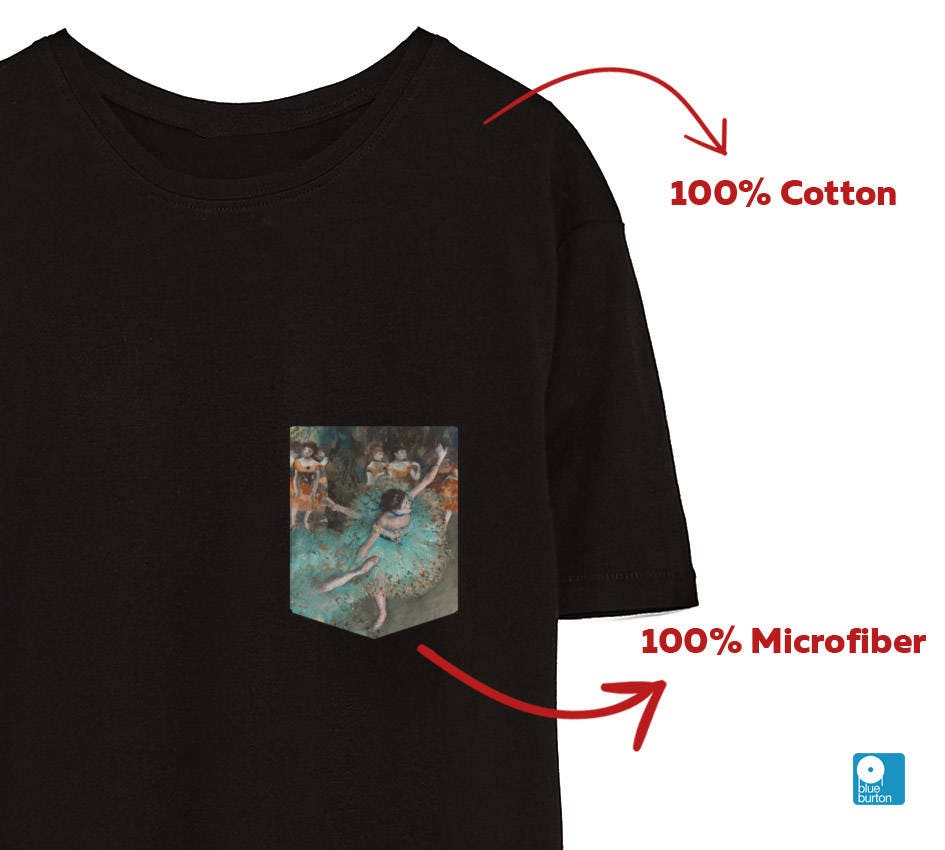The image displays a black, round-neck, short-sleeve t-shirt against a white background. However, only the right sleeve and the upper half—from the neck to the middle—is visible. The t-shirt features a small, pocket-sized design towards the right side. This design includes an animated scene with several people in red and a lady twirling in a blue ballerina outfit with a circular skirt. 

Two red arrows are superimposed on the image, both curving towards the right side. The first arrow stretches from the shoulder of the t-shirt and points to the text "100% cotton," written in the same red color as the arrow. The second arrow initiates below the ballerina design and also curves to the right, pointing towards the text "100% microfiber," again in red. Both arrows and text highlights appear to emphasize the fabric composition of the t-shirt.